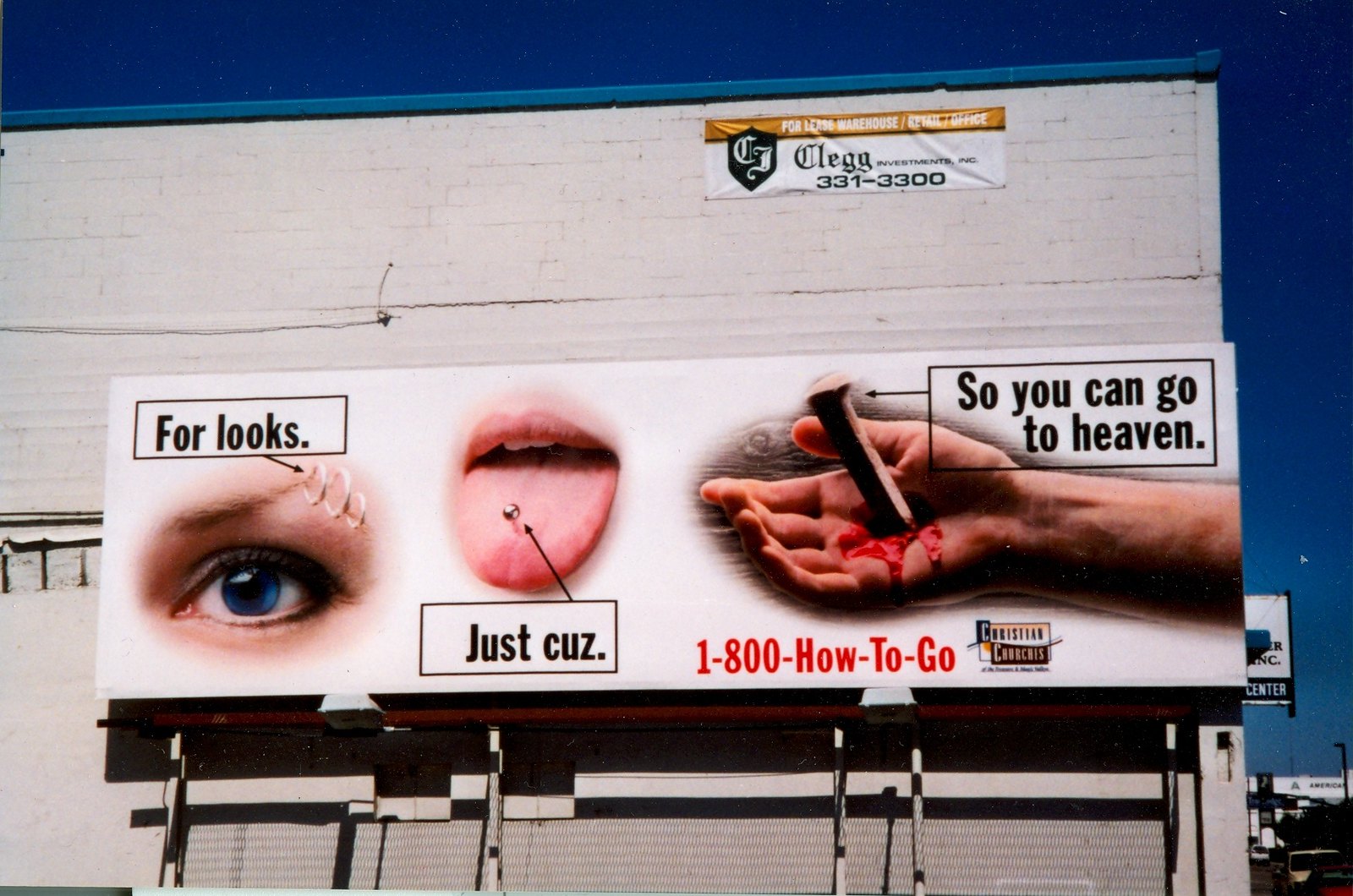The image is a photograph of the side of a white, brick or stone building with a blue rain gutter at the top. The dark blue sky serves as the backdrop, and a sign near the top reads "Clegg Investments, Inc." with contact details for leasing a warehouse, retail, or office space. In front of the building, there is a detailed advertisement billboard. The billboard is predominantly white with various graphic elements. 

At the top of the billboard, there's the caption "For Looks" pointing to an eye with three piercings on the eyebrow. Below that, the words "Just Cause" point to a mouth sticking its tongue out, with a tongue piercing clearly visible. To the right side of the billboard, there is a graphic of an outstretched hand with a metal stake driven through the palm, along with blood, under the caption "So You Can Go to Heaven." At the bottom in red letters, it reads "1-800-How-To-Go" with an additional graphic that says "Christian Churches."

This advertisement appears to contrast body piercings with Christian salvation, suggesting that avoiding body modifications is linked to going to heaven.